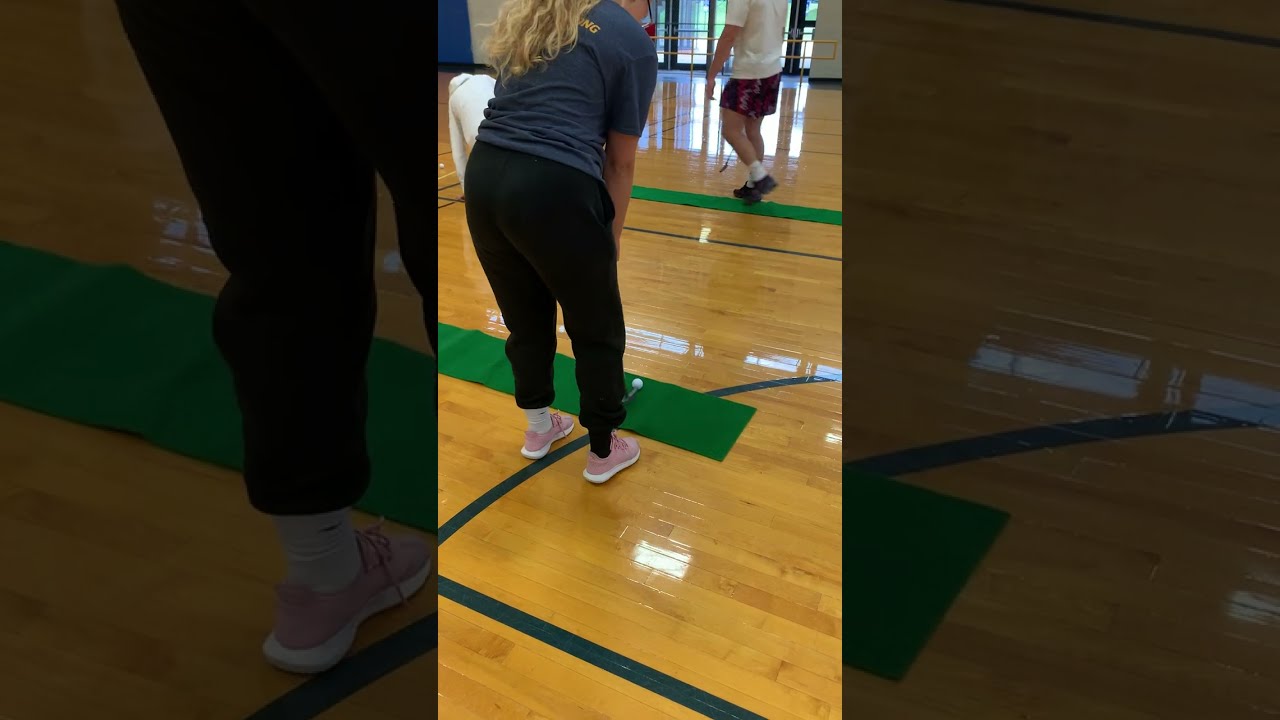The image depicts an indoor scene at a sports gym with wooden flooring marked with blue lines typically used for basketball courts. In the foreground, a woman with long, wavy blonde hair is slightly bent over, putting a small white golf ball on a green felt rectangular mat. She wears a navy blue t-shirt with yellow lettering partially visible ("ING"), black sweatpants, and pink sneakers with white and black socks. To the rear, another individual, whose head is not visible, is dressed in a white short-sleeved shirt, purple and pink shorts, and black shoes, similarly engaged in putting a golf ball on their own green felt mat. The overall atmosphere reflects a training session, utilizing these narrow green strips for practicing putting indoors.